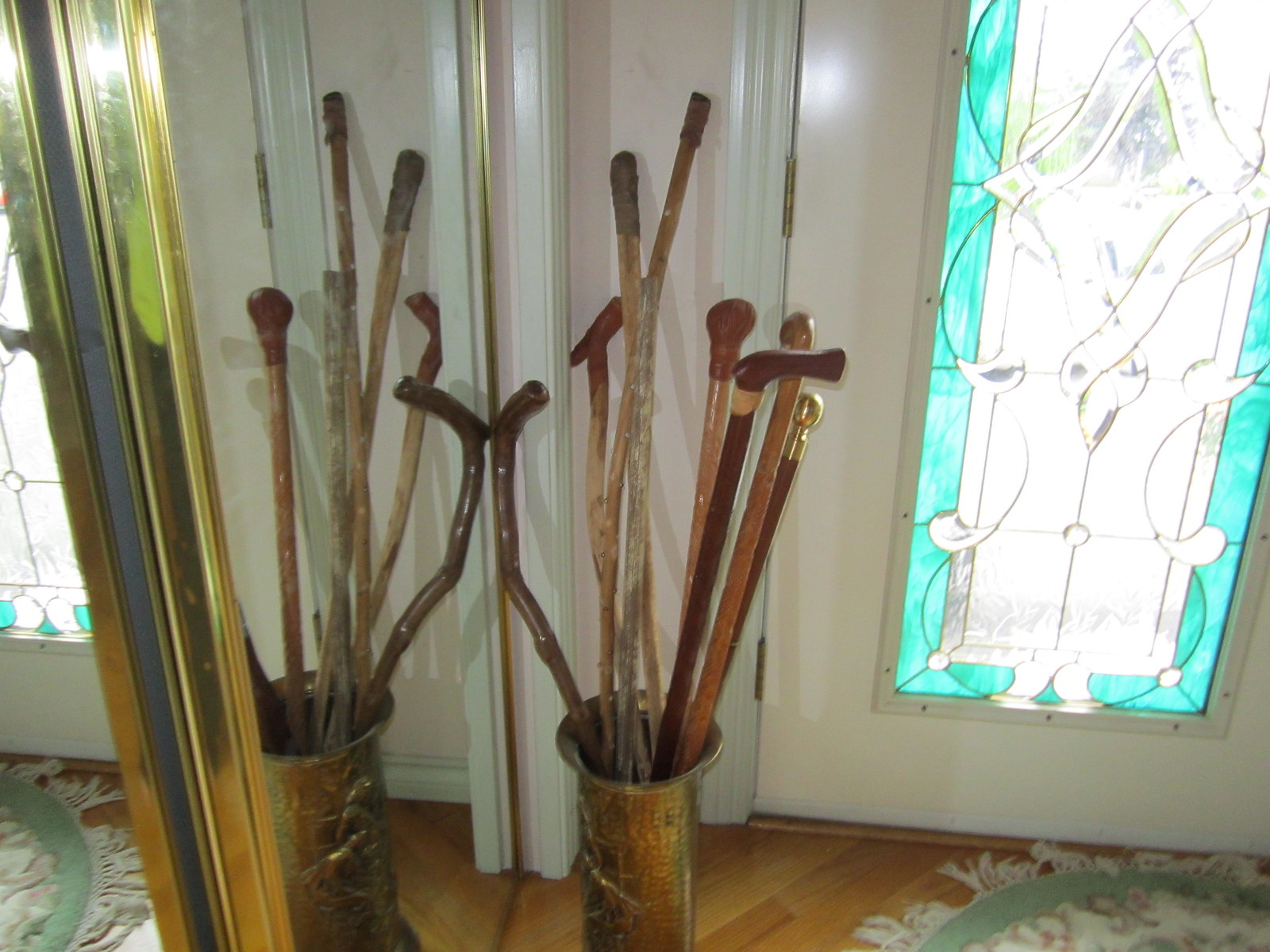The photograph captures the inner foyer of a home, with a striking front door adorned with an elaborate stained glass window in white and aqua blue. Sunlight streams in through the door, highlighting its intricate design with a turquoise frame and a clear middle section. The foyer features hardwood floors and a doormat near the door. To the left of the door, a set of seven or eight wooden walking sticks, each with unique handles and varying shades of brown, are stored upright in a yellow copper vase. Adjacent to this is a mirror framed in gold, which reflects the image of the walking sticks. A glimpse of a circular rug with a green border and white fringes is visible on the wooden floor. The scene exudes a warm, welcoming atmosphere with a charming blend of decorative details.